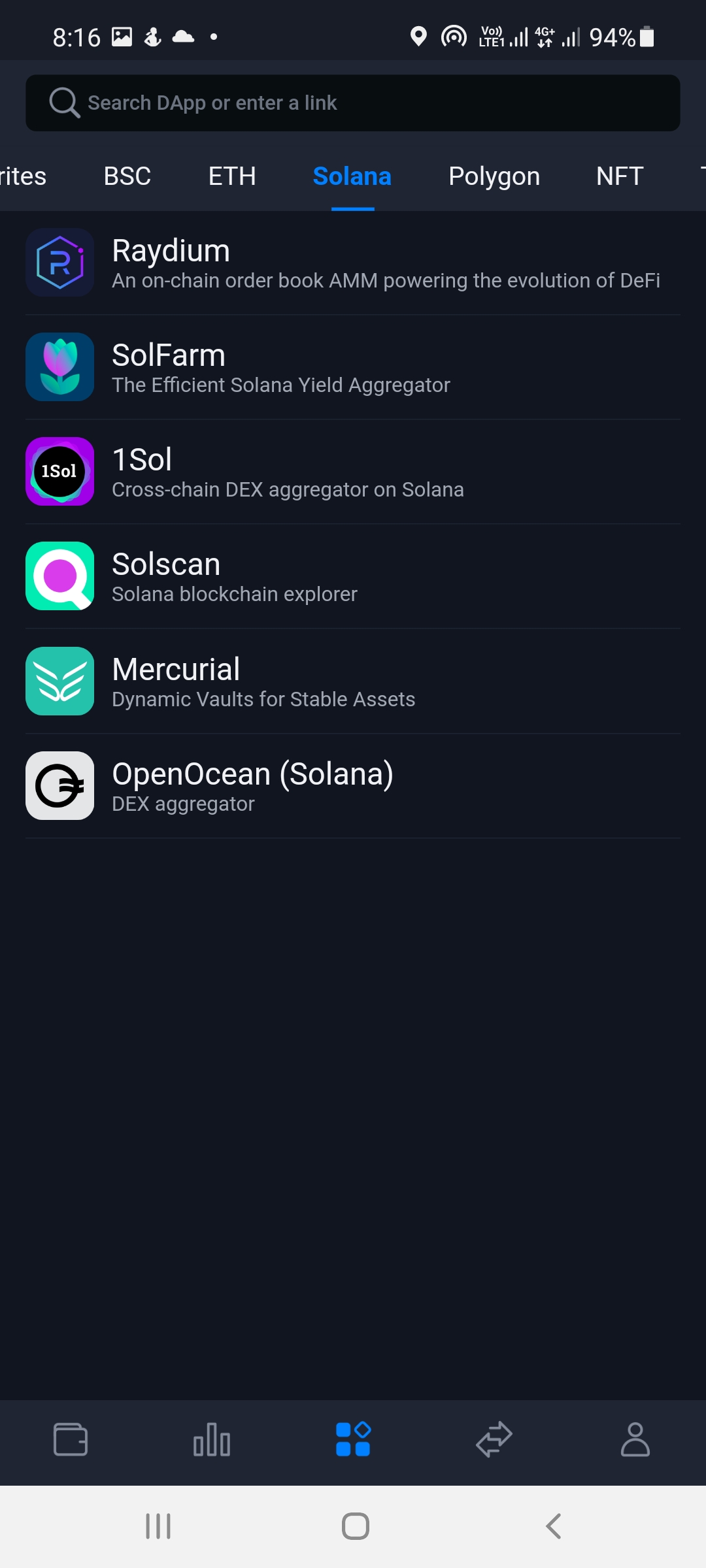A detailed screenshot of a smartphone displaying a cryptocurrency trading application, specifically set to the Solana blockchain category. The status bar at the top shows the time as 8:16, along with various icons including a photo gallery shortcut, a cloud saving symbol, a location indicator, a service indicator, a 4G network status symbol, and a nearly full battery at 94%. Just below the status bar, there is a search bar where users can search for decentralized applications (dApp) or enter a specific link, with the search icon situated on the left side.

Immediately below the search bar are buttons for selecting different blockchains, namely Binance Smart Chain (BSC), Ethereum (ETH), Solana, Polygon, and NFTs. The Solana button is currently selected. Subsequently, a list of available cryptocurrencies within the Solana category is displayed: 
1. Radium - an on-chain order book Automated Market Maker (AMM) supporting DeFi evolution.
2. Solfarm - an efficient yield aggregator for Solana.
3. OneSol - a cross-chain Decentralized Exchange (DEX) aggregator on Solana.
4. SolScan - a Solana blockchain explorer.
5. Mercurio - a Dynamic Vault for stable assets.
6. OpenOcean - a Solana DEX aggregator.

At the bottom of the application interface, there are navigation buttons for Wallet, Charts, Favorites, Transfers, and an account user icon. Additionally, the smartphone's standard UI buttons for minimizing, opening applications, and returning to the previous screen are located at the very bottom of the display.